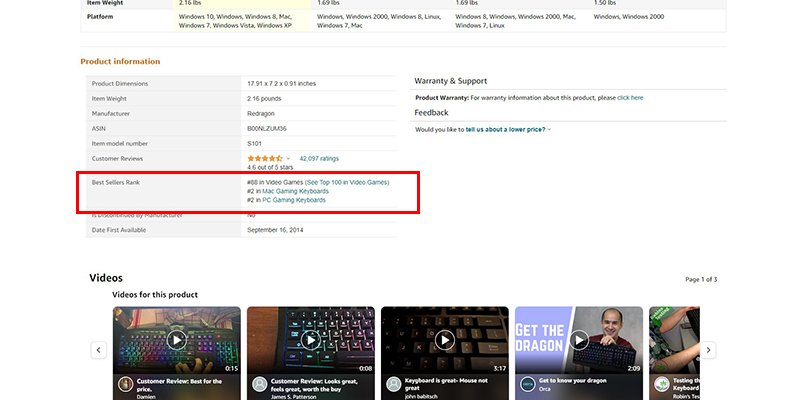This is a detailed screenshot captured from an Amazon product page, specifically focused on the product information section. The visible portion of the page provides key details including the product dimensions (17.91 by 7.2 by 0.91 inches) and item weight (2.16 pounds). The manufacturer is listed as Red Dragon, and the ASIN number, as well as the item model number, are partially visible. The product has an impressive customer rating of 4.6 out of 5 stars, based on 42,097 reviews. A red box highlights its bestseller rank, where it stands at #68 in the Video Games category, and notably ranks #2 in both Mac Gaming Keyboards and PC Gaming Keyboards categories. The date first available is mentioned as September 16, 2014. Below this section, there are several thumbnail videos related to keyboards, which are horizontally scrollable from left to right.